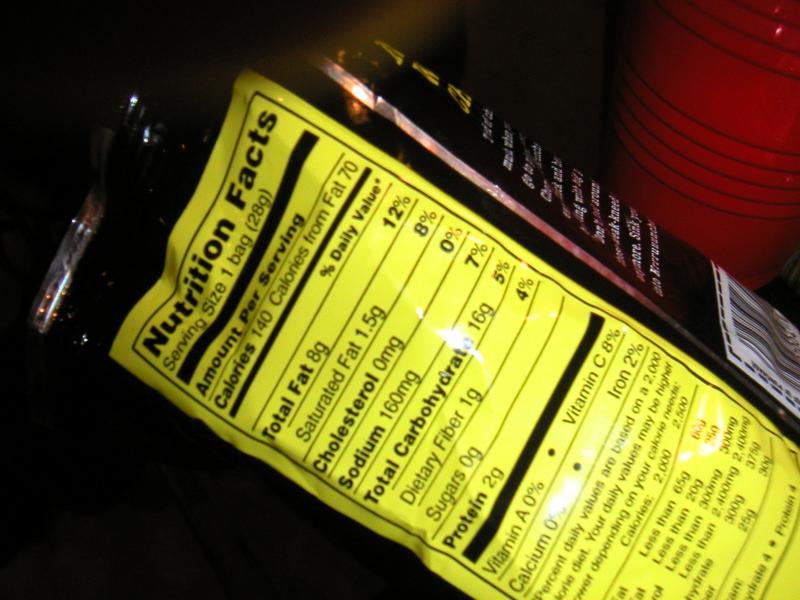A detailed image caption could read:

"This image captures a close-up of a product label adhered to a black packaging bag, which is tilted slightly to the left. Prominently featured on the label is a vertical rectangular yellow section displaying the Nutrition Facts. The text on the right side of the package includes a UPC barcode. Above the barcode, the white text on the yellow background details the nutritional information: Serving size - one bag, Calories - 140, Calories from fat - 70. Horizontal black lines separate this data, followed by a detailed list of nutrients and their respective percentages. Further nutritional details and percentages are listed below another black horizontal line, with additional text rounding out the bottom of the label. The entire scene is set against a black background, with a red cup positioned in the lower right-hand corner of the frame."